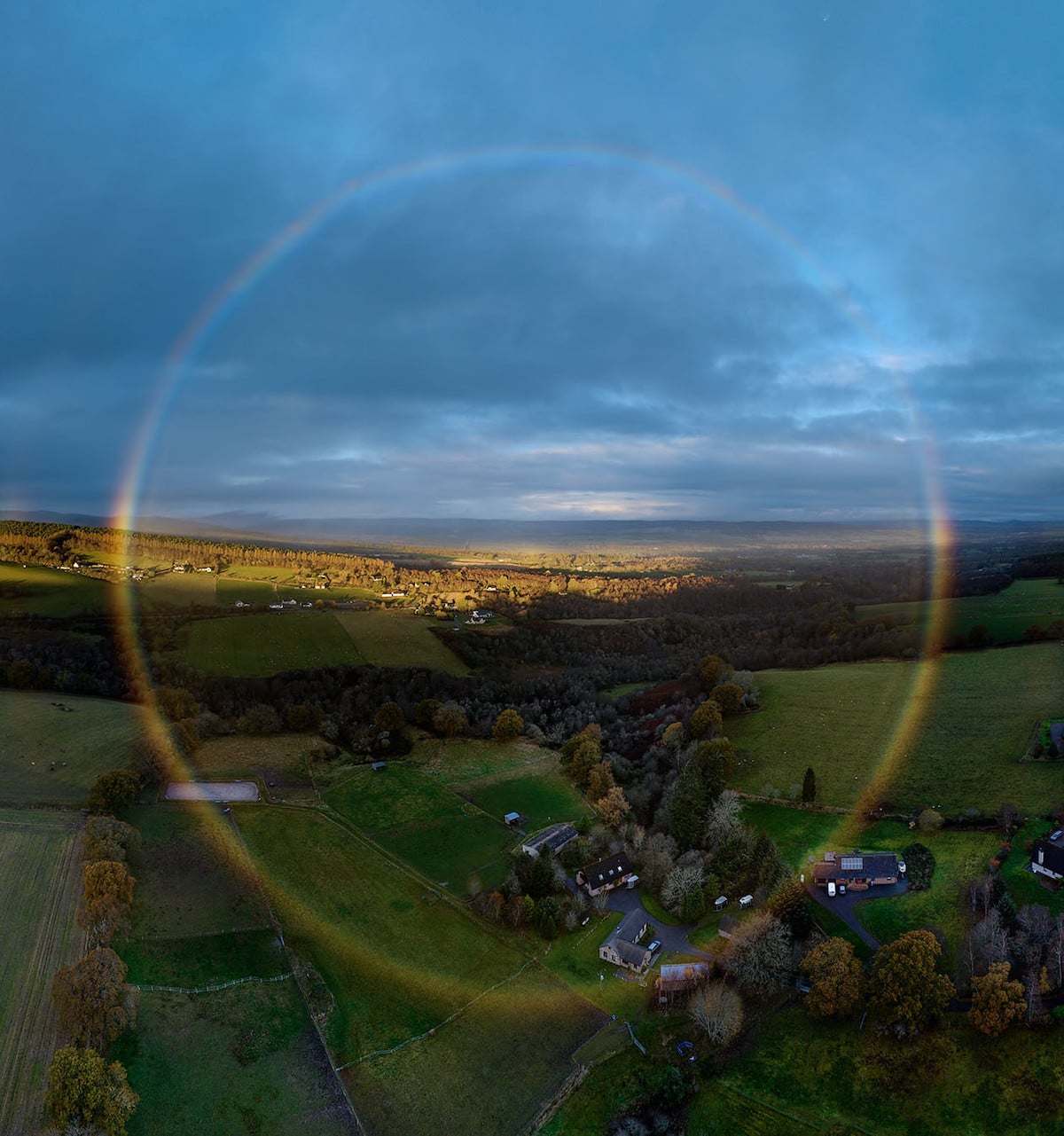This color photograph, taken in portrait orientation, presents an aerial view of a rural coastal community. Toward the bottom center-right, clusters of farmhouses are nestled among various shades of green pastures and fields, demarcated by fences and roads. The landscape features a mixture of green and brown hues, with trees along the fields displaying autumnal shades of orange and yellow. In the distance, a village or town is visible, framed by a horizontal sliver of the grayish-blue ocean on the horizon. The sky above is overcast with dark gray clouds, though a portion of the village or town is illuminated by a soft light, suggesting it is either morning or dusk. A distinct circular ring of light, possibly a special lens effect, radiates from the center of the photograph, adding a unique visual element. The scene is set against a backdrop of green mountains, completing this realistic and detailed depiction of the tranquil, rural landscape.